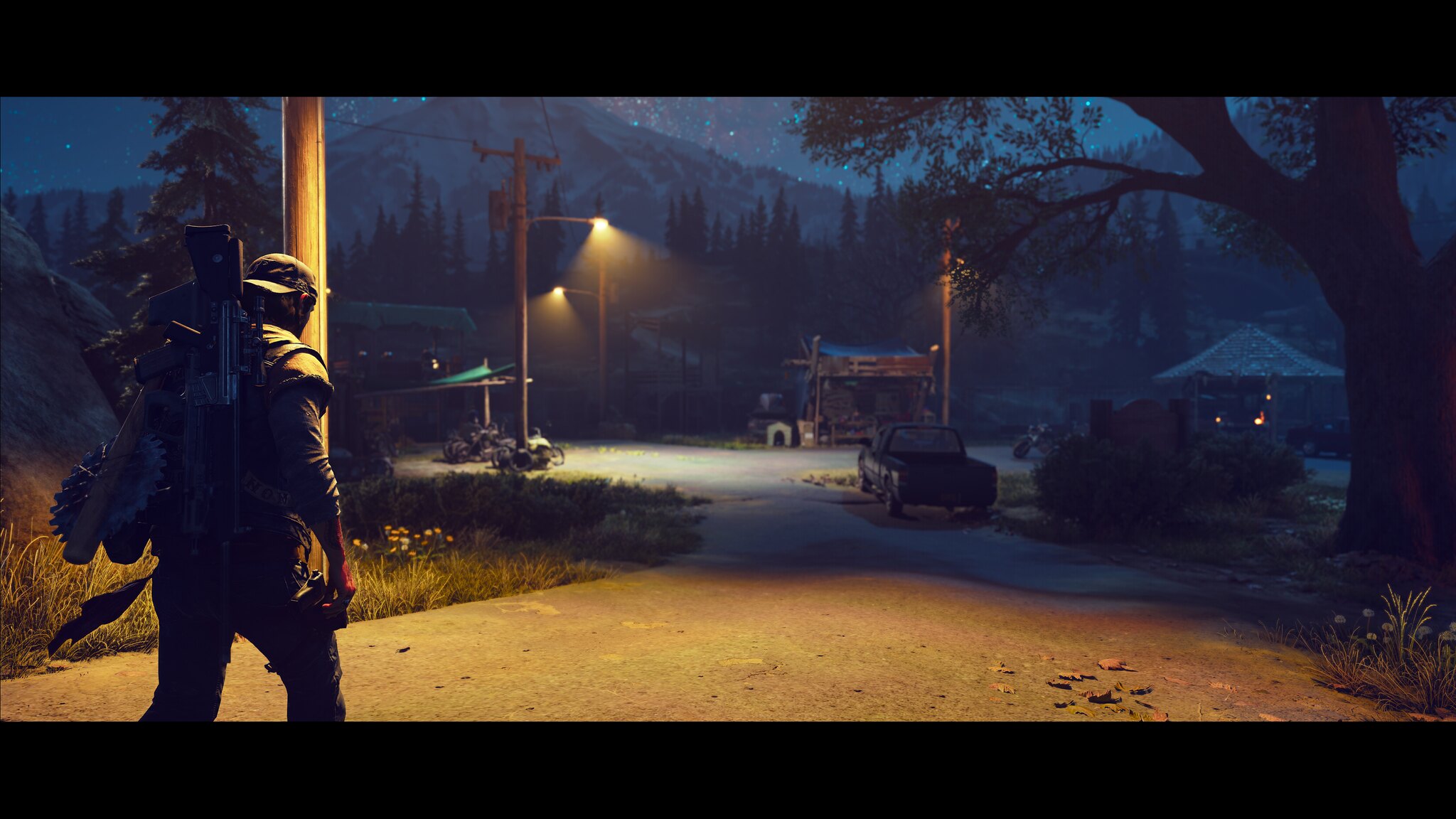The image is a detailed and atmospheric illustration set outdoors at night, depicting a rugged, mountainous landscape under a starry blue sky. A high mountain peak, dotted with spruce-like trees, dominates the background, while a series of rustic buildings, including a small shack and another cabin-like structure with three illuminated windows, nestle against the mountainside. Alongside the structures, a dirt road winds its way illuminated by tall wooden streetlights, leading towards the foreground where a figure walks away from the viewer.

This figure, possibly a hiker, camper, or military man, is caught mid-stride on the road. He has a rugged appearance, wearing wrinkled clothing that includes a three-quarter length shirt, a vest, camouflage pants, and a backpack laden with several weapons. His cap is turned backwards, and there appears to be a fish attached to his left hip. A motorcycle and a pickup truck are parked near the buildings, adding to the scene’s rustic, remote feel.

The ambiance is further enhanced by patches of grass, weeds, and flowers in the shadows, contributing to the serene yet mysterious night-time setting. The composition skillfully combines elements of wilderness adventure and solitude, creating a compelling narrative within the confines of a wide and narrow horizontal frame.